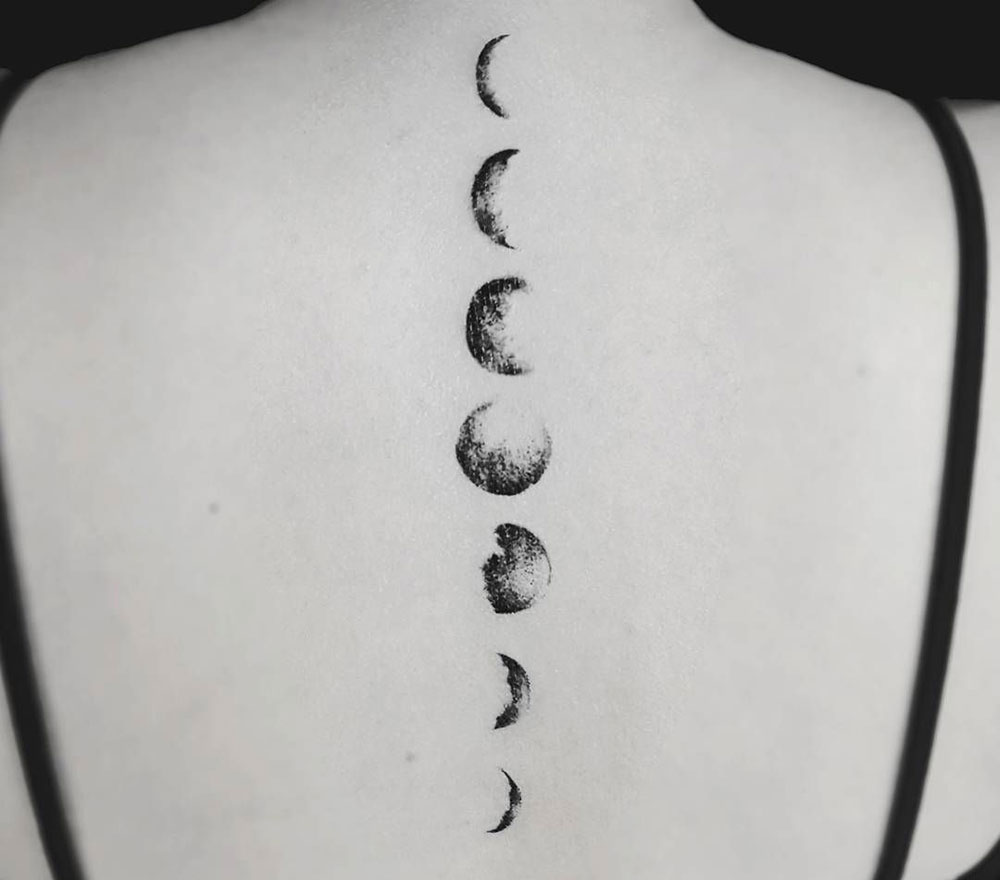This black and white photograph, seemingly from an earlier era, captures a close-up of a woman's pale back adorned with an intricate tattoo of the moon's phases. The woman is dressed in a black strapless top, visible through two thin straps on her shoulders and a horizontal strap across her upper back. The focal point is the vertically arranged moons, beginning at her mid-back and extending to her neckline. The tattoo features seven phases: starting with crescents at the bottom facing left, progressing through quarter and half moons, with a full moon at the center, and concluding with crescents at the top facing right. The monochromatic tones accentuate her fair skin and the detailed lunar artwork.